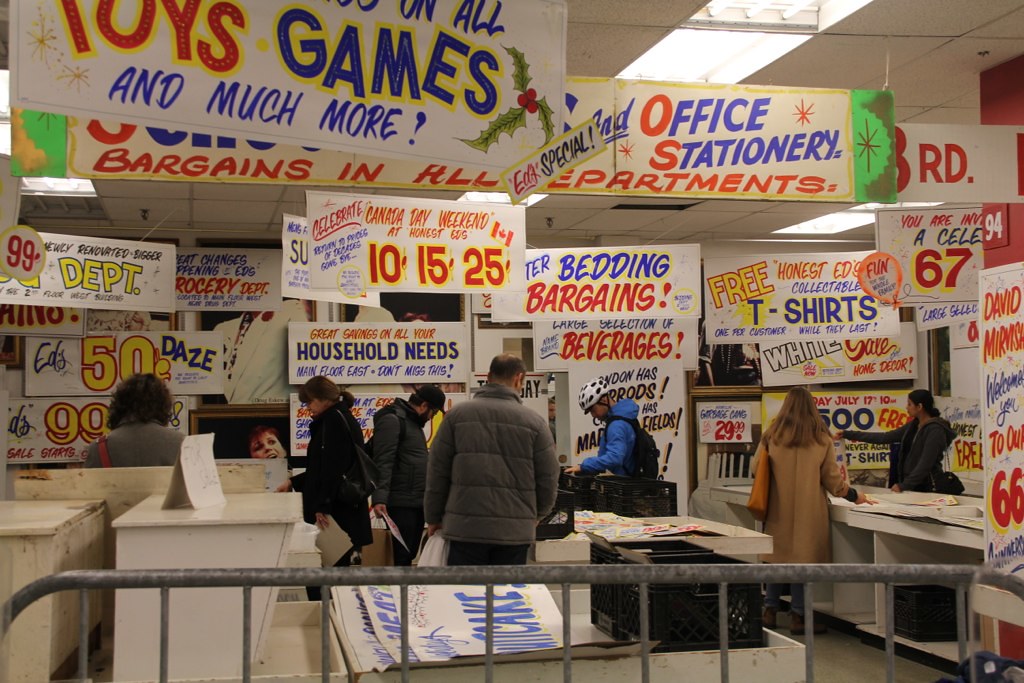This photograph captures the interior of a store, taken from behind a gray metallic gate visible at the bottom of the image. Beyond the gate, several desks or counters are organized, some of which have signs attached to them. In front of the gate, there's a black plastic crate. Various signs hang from the ceiling and along the sides of the store, advertising toys, games, and more, with many displaying prices. One notable sign is positioned in the upper left corner, partially entering the frame. The scene is bustling with colorful signage that adds vibrancy to the commercial setting.